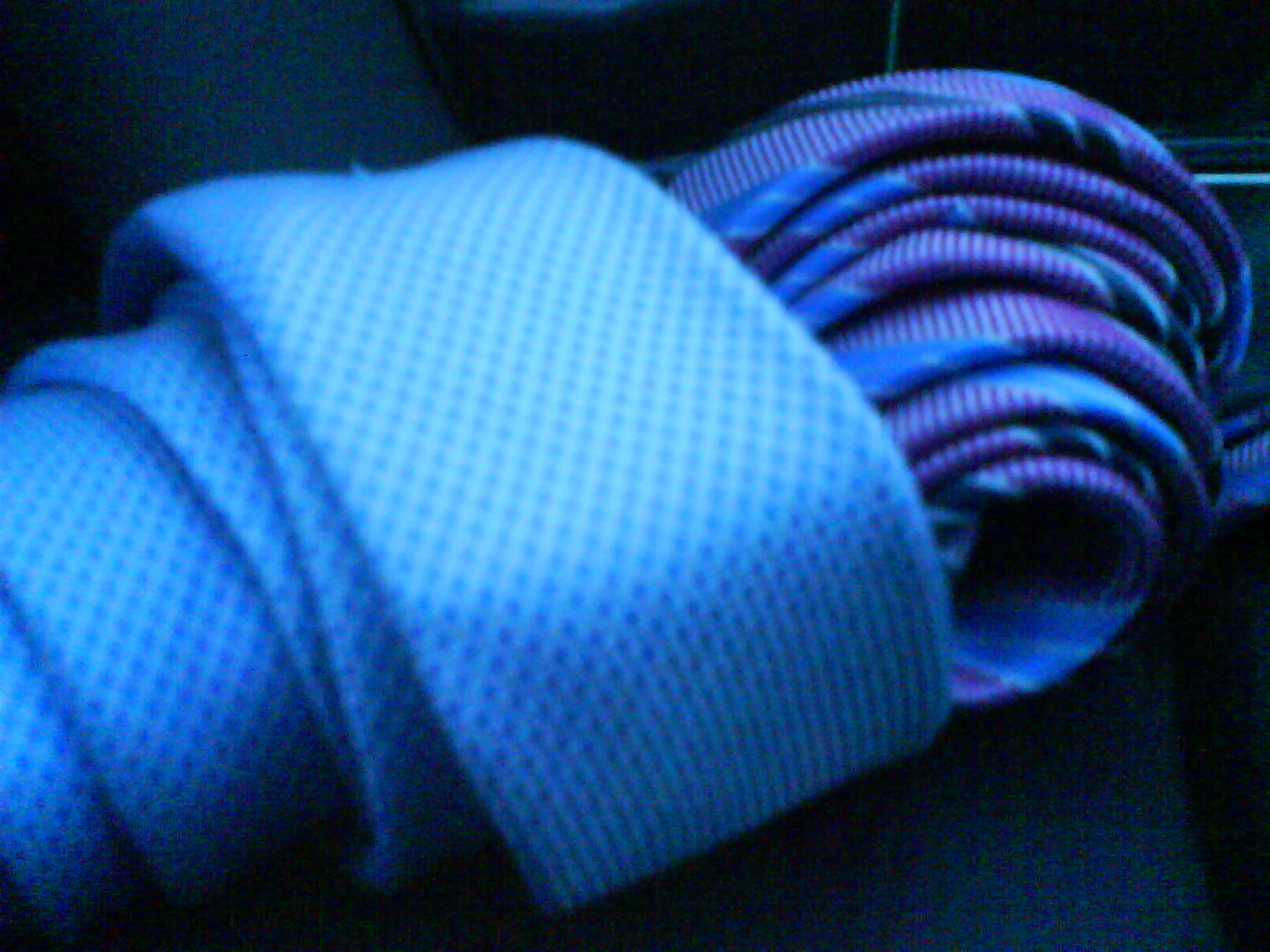This is a detailed close-up image of two intricately rolled neckties resting on a dark navy blue fabric surface, with a blue-tinted reflection. The tie on the left, positioned towards the bottom, features a simple pattern of blue and white diamond dots arranged diagonally. This tie, coiled into five distinct rolls, wraps around itself beginning from the left corner and extending slightly past the middle. The tie on the right, positioned more towards the upper right corner, consists of eight rolls, which progressively increase in size. This tie boasts a more complex color palette, including light blue, silver, stripes of red with a subtle white pattern, and possibly dark blue or dark silver elements. Each rolled tie maintains a precise cylindrical form, showcasing both the intricate patterns and textures of the fabric in pristine condition. The dark navy blue background enhances the contrast and highlights the vivid details of the neckties.